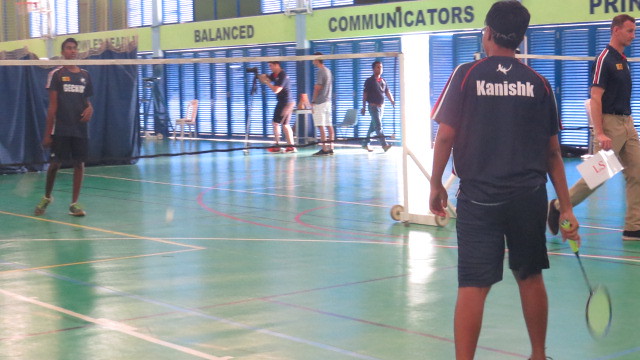This image captures an indoor badminton court situated in a gymnasium with a green floor marked by purple and white lines. The court is separated from the rest of the gym by blue curtains, and the backdrop reveals large windows letting in daylight. Two men stand ready to play; the player closest to the camera wears a blue shirt with "Kanishk" printed on it, paired with a blue hat and white shorts, and he grips a badminton racket. Across the net, another man in a similarly colored shirt and white shorts prepares to engage. The gym walls are adorned with yellow banners that read "balanced communicators," and various individuals walk in the background. Notably, one man sets up a camera on a tripod while another carries a paper labeled "LS" and an LS bag. Overall, the scene depicts the anticipation and activity surrounding a friendly yet competitive badminton game.